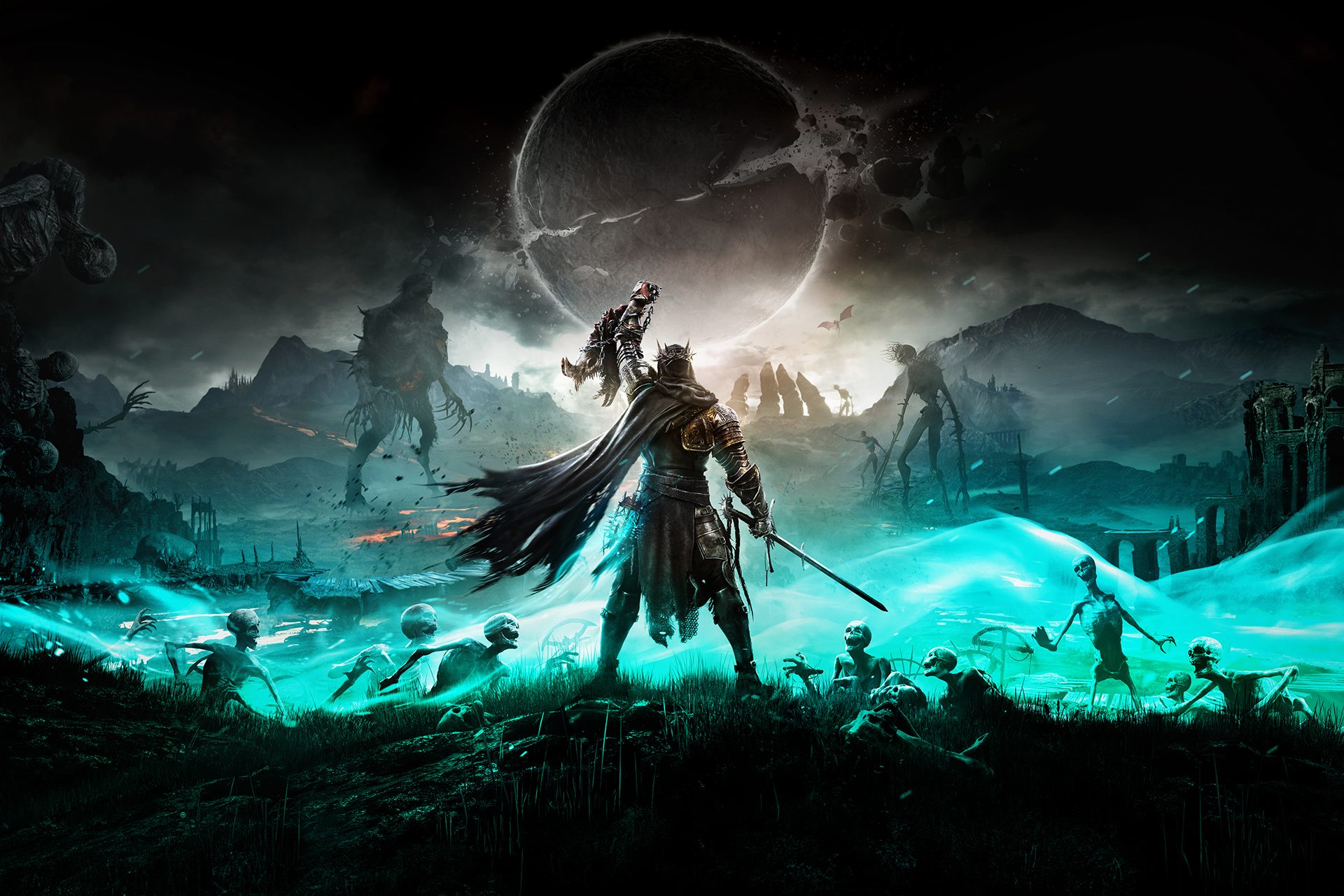In this captivating fantasy scene, set against a moonlit night, a warrior king stands resolute at the center of a fragmented, surreal battlefield. Dressed in metallic armor and draped in a flowing cape, he faces away from us, his long sword held firmly in his right hand while he lifts his left arm defiantly, clutching an object or perhaps a fallen creature above his head. His appearance is crowned, indicating his regality. The landscape stretches out in a panoramic format, with dark skies occupying the top and bottom thirds of the frame, adding an ominous tone to the piece.

The foreground reveals a menacing legion of skeletons, possibly zombies, slowly rising from the earth and bathed in an eerie aqua-colored light. This chilling illumination offers stark contrast against the otherwise dimly lit surroundings. Adding to this unsettling atmosphere, towering robotic figures loom in the distance, seemingly advancing toward the king's presumed kingdom or territory. The environment is dotted with small fires and appears desolate but charged with tension.

Towards the background, dark hills and mountains shroud the horizon, while a body of light blue water separates the chaotic foreground from these distant ominous shapes. A colossal creature with elongated fingers can be seen to the left, alongside other sinister entities that populate this alien terrain. Central to the sky is a celestial event, possibly a solar eclipse, casting an otherworldly glow over the entire landscape. This intricately detailed scene weaves a narrative of defiance and despair, capturing a critical moment in an epic, fantastical struggle.